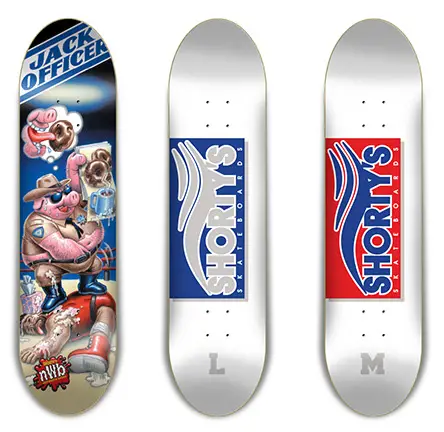The image features three illustrated skateboard decks against a bright white background. On the far right, there's a silver-colored skateboard adorned with a large, red decal reading "Shorty's Skateboards" and an 'M' toward the bottom. Next to it, another silver skateboard mirrors this design but with a blue decal and an 'L' at the bottom. Both decals feature the Shorty's logo, which resembles stacked wavy skateboard ramps. The deck on the far left stands in stark contrast with a vividly detailed, Garbage Pail Kid-style illustration. This skateboard displays a cartoonish, anthropomorphic pig dressed as a sheriff, complete with a tan uniform, badge, hat, and sunglasses. The pig, with his belly hanging out and one trotter hand down in his pants, stands on a prostrate wrestler. The pig's other hand holds a tray with two doughnuts and a cup of coffee, while a thought bubble shows the pig's tongue licking chocolate glaze off a doughnut. The scene is captioned "Jack Officer," with a box of tissues and suspicious white globs adding a crude element to the depiction. The acronym "NWB" appears in the bottom left of the illustration. The detailed, contrasting designs offer a vivid and eclectic mix of skateboard art.